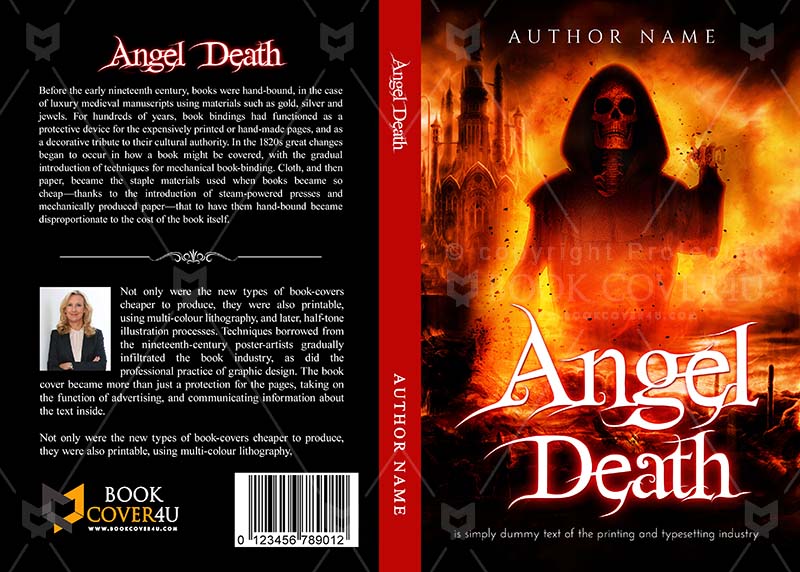This image depicts the complete jacket for a book titled "Angel Death," showcasing both the front and back covers, as well as the spine, in a single view. The left side is the back cover, featuring a black background with striking white text bordered in red, displaying the title "Angel Death." Below, there's a detailed explanation about the evolution of book binding from luxurious, hand-bound medieval manuscripts adorned with gold, silver, and jewels to the more mechanically bound and affordable books of the 19th century. Midway down the back cover, a white ornate dividing line separates the historical text from a small black and white photograph of a blonde woman dressed in a suit shirt, accompanied by additional text about the advancement of book covers through multicolored lithography and halftone illustration processes. 

At the bottom left, a black and orange icon resembling an open book accompanies the URL "www.bookcover4u.com," while the UPC barcode resides in the bottom right corner. The spine of the book is bordered in red, displaying the title "Angel Death" in white text, along with the author's name.

On the right side, the front cover captivates with an intense graphic design featuring a castle engulfed in fiery orange flames in the background. Dominating the foreground is an eerie human skeleton cloaked in a black hoodie, lifting its right hand. The title "Angel Death" and the author's name appear at the top and bottom in white text, standing out against the dynamic and dramatic fiery backdrop. This book cover skillfully merges historical homage and modern design, capturing the attention through both visual and textual storytelling.